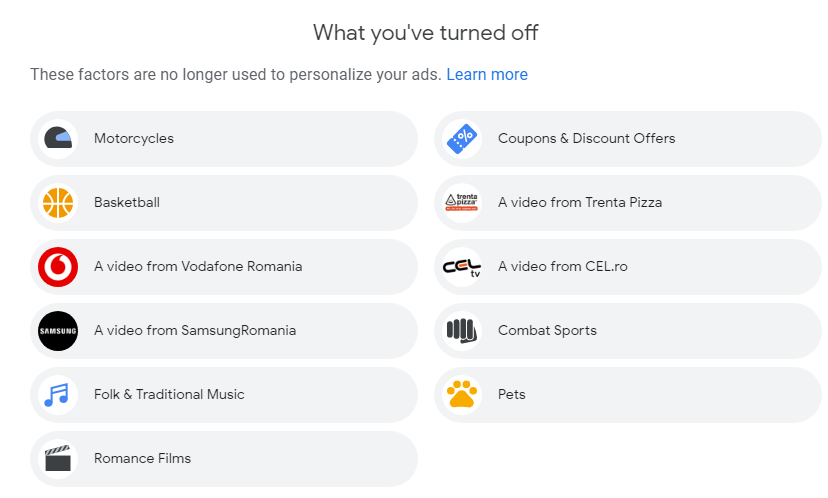A screenshot displays a list of categories and items that have been deactivated for ad personalization. The categories shown in the list include motorcycles, basketball, and a video from Vodafone Romania (spelled out as V-O-D-A-F-O-N-E). Additionally, a video from Samsung Romania is listed, with both 'Samsung' and 'Romania' capitalized. Other categories in the list are folk and traditional music, romance films, coupons and discount offers, a video from Trentapizza (spelled out as T-R-E-N-T-A), a video from Celdoro (capitalized as C-E-N-L), combat sports, and pets. The words "more and more" are highlighted in blue.